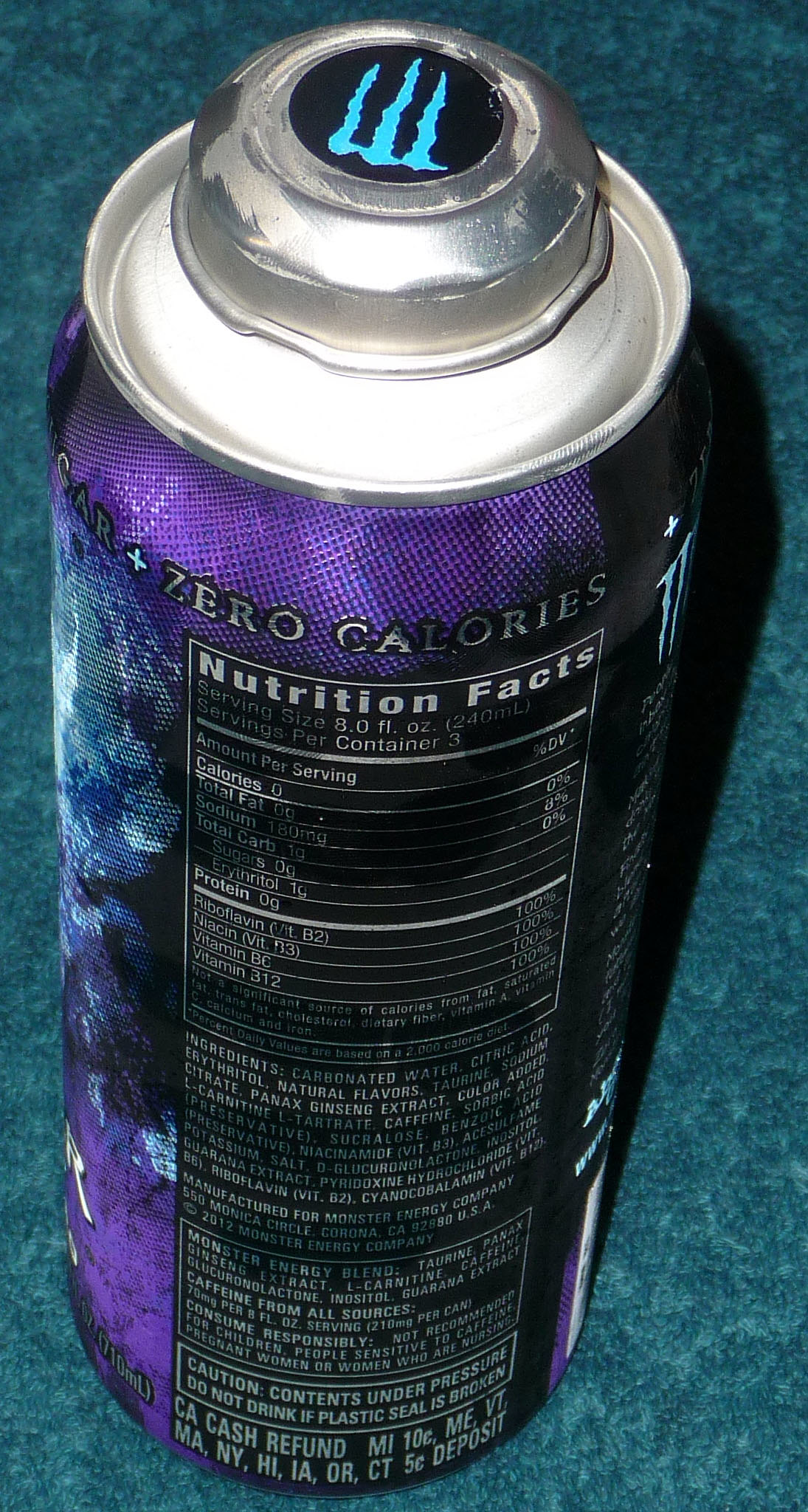This image is a detailed photograph of a Monster energy drink can, predominantly showcasing its back side. The can itself is a rich, dark purple color with a black label area on the left side featuring light blue designs that extend around to the front. The can is positioned on a table with a marbled navy blue and light blue background.

At the top of the can, there's a silver top with a twist-off cap that is a darker silver with a black circle and a light blue "M" for Monster. The can prominently displays "Zero Calories" at the top back in gray and black letters. Below this, there's a long rectangular area containing the nutritional facts in white lettering on a black background. Adjacent to this section, there is a design with bluish-black tones further accentuating the can's aesthetic.

Additionally, the can includes another blue Monster symbol at the top right, a barcode at the bottom right corner, and a detailed nutritional chart with ingredients listed underneath the primary nutritional facts, all on a black and white label. The can's design, combining blue, purple, black, and light blue elements, offers a visually striking and dynamic appearance.